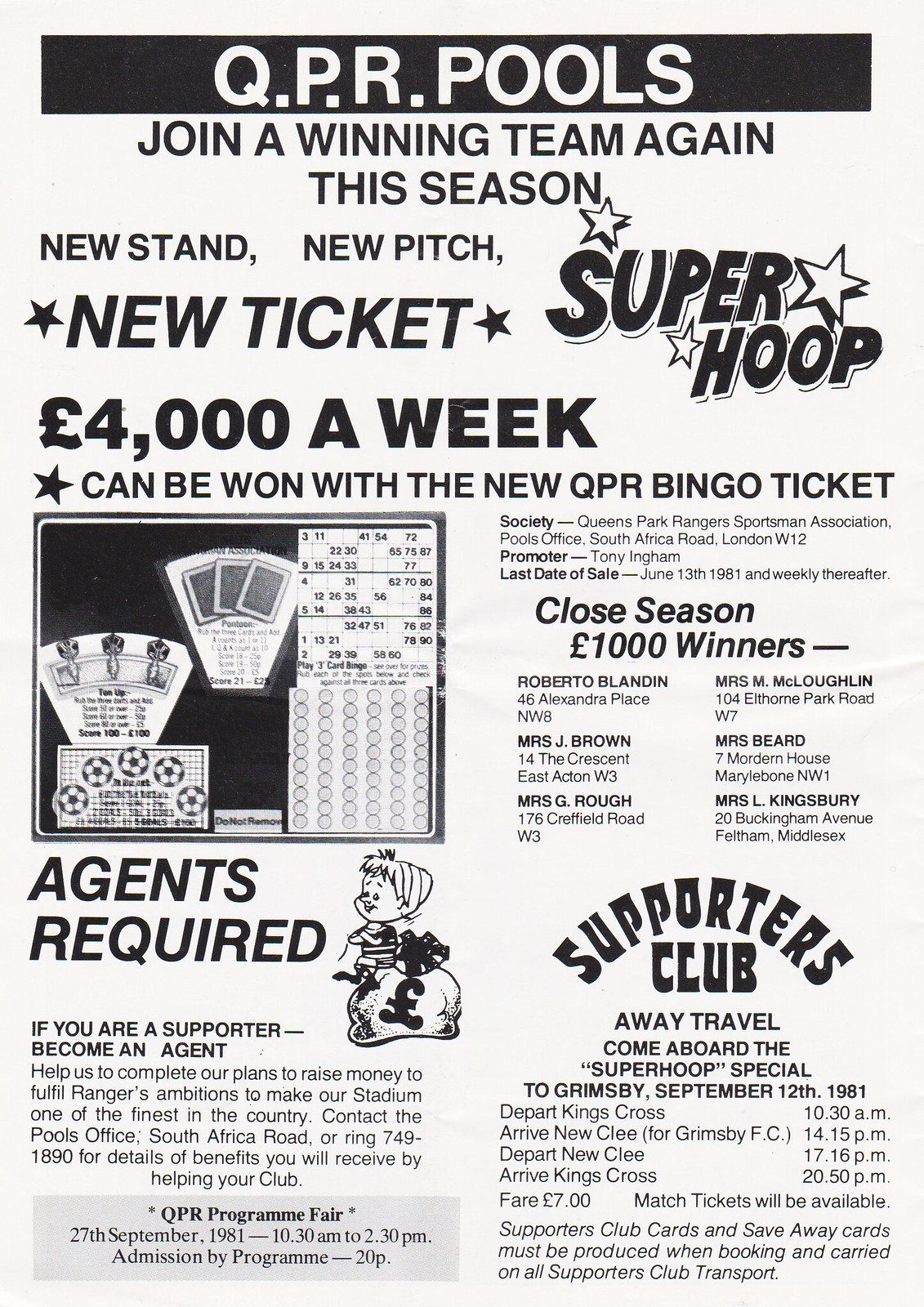The image is a vertically aligned, black-and-white flyer that serves as an advertisement for Q.P.R. Pools. At the very top, there is a black rectangular bar with white all-caps text that reads "Q.P.R. POOLS." Below this, in black text, the flyer invites readers to "Join a winning team again this season." Further down, the text continues in black, highlighting "New stand, new pitch," followed by "NEW TICKET" in large, bold, all-caps text with stars on either side. To the right, in bubble letters with several stars around it, the words "SUPER HOOP" stand out in bold black text. Directly below, it states "4,000 pounds a week" in large, bold text, explaining that this amount "can be won with the new Q.P.R. bingo ticket." Additional smaller text details that supporters can become agents to assist in raising money for Q.P.R.'s ambitions to enhance their stadium, advising to contact the Pools Office at South Africa Road, London W12, or ring 749-1890 for more details. There is also a mention of a supporters' club away travel event, specifically a "Super Hoop Special" to Grimsby on September 12th, 1981. Images on the flyer include a depiction of some playing cards, soccer balls, and a betting card.